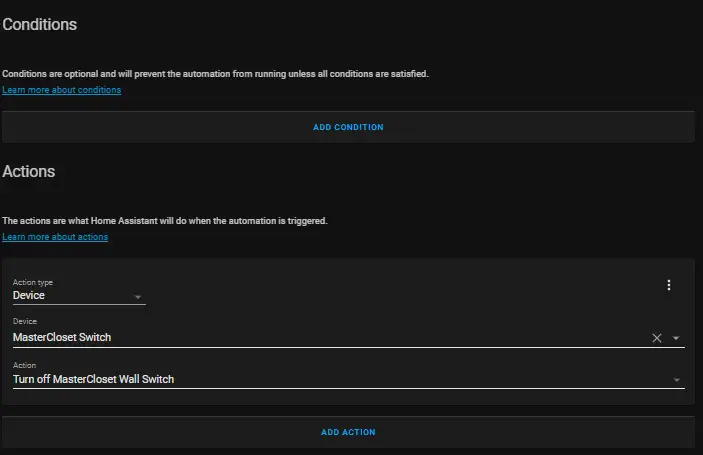Here is a cleaned-up and detailed caption based on the provided voice description:

"The image depicts a user interface for setting up home automation. At the top left, a grey background section labeled 'Conditions' explains that these are optional criteria which must all be met to allow the automation to run. A button labeled 'Add Condition' is present underneath. Below this section, the 'Actions' portion describes what actions the home assistant will perform when the automation is triggered. Users can learn more about conditions and actions through links provided.

Currently, the action type is set to 'Device' with a down arrow indicating a dropdown menu for other options. To the right, three small dots represent additional settings. A button labeled 'Device Master Closet Switch' is selected, with an 'X' and an arrow for editing or removing the selection. The specified action is 'Turn off Master Closet Wall Switch,' accompanied by another arrow for more options.

At the bottom, there are buttons to 'Add Action' and 'Add Condition,' both with 'Learn More' links in blue text. Selections with arrows and underlines indicate interactive elements throughout the interface."